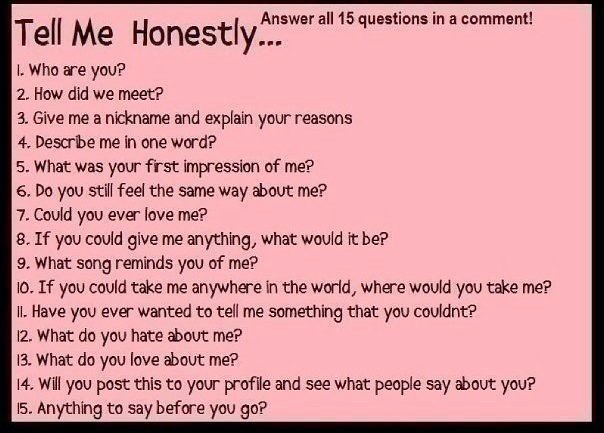The image is a graphic design with a pink rectangle background bordered by a thin black rule. It looks like a screenshot from social media, likely Facebook. Centered on the image is black text with a headline that reads, "Tell me honestly..." followed by "Answer all 15 questions in a comment!" The text is aligned to the left and lists 15 numbered questions: 1. Who are you? 2. How did we meet? 3. Give me a nickname and explain your reasons. 4. Describe me in one word. 5. What was your first impression of me? 6. Do you still feel the same way about me? 7. Could you ever love me? 8. If you could give me anything, what would it be? 9. What song reminds you of me? 10. If you could take me anywhere in the world, where would you take me? 11. Have you ever wanted to tell me something that you couldn't? 12. What do you hate about me? 13. What do you love about me? 14. Will you post this to your profile and see what people say about you? 15. Anything to say before you go? The graphic design and typography style aim to engage users in a series of reflective and personal questions.